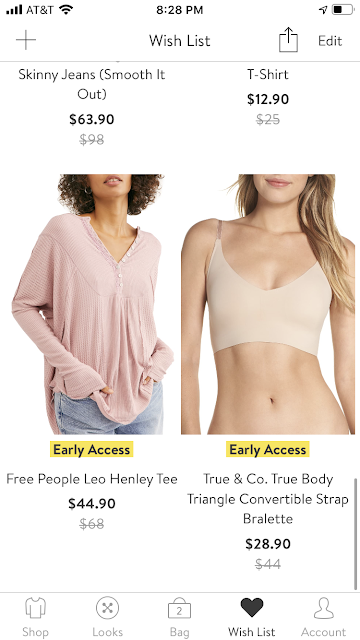This appears to be a detailed screenshot of a mobile shopping app focused on clothing. 

**At the top-left corner**, there are icons indicating a signal, the carrier labeled as "AT&T," and a Wi-Fi symbol. Centered at the top, the time is displayed as "8:28 PM." To the right of the time, there is an arrow pointing upwards and a battery icon showing a half charge.

**Below the status bar**, the header section includes a "+" sign on the left, the word "Wishlist" in black text centered, and a box with an upward arrow followed by the word "Edit" in black text on the right.

**In the main content area**, there are two columns showcasing items:
- **Left column**:
  - "Skinny Jeans (Smooth It Out)" priced at $63.90, with the original price of $98 crossed out.
  - Below this text, there is an image of a woman with dark curly hair and a brown complexion, wearing a long-sleeve pink shirt and blue jeans.
  - Underneath her image, there's a yellow box with black text reading "Early Access" and "Free People Leo Henley Tee" priced at $44.90, with the original price of $68 crossed out.

- **Right column**:
  - A t-shirt priced at $12.90, with the original price of $25 crossed out.
  - Below this, there's an image of a woman with a pale complexion and long blonde hair, wearing a halter top bikini.
  - Underneath her image, a yellow box with black text says "Early Access" and "True & Co True Body Triangle Convertible Strap Bralette" priced at $28.90, with the original price of $44 crossed out.

**At the bottom of the screen**, there are five icons indicating different sections of the app:
- On the left, a shirt icon labeled "Shop."
- A circle with an X icon labeled "Looks."
- A central bag icon with the number "2" indicating items in the cart.
- A heart icon in black labeled "Wishlist."
- A silhouette of a face with a count, presumably for account-related actions or notifications.

This screenshot captures a well-organized interface showcasing various fashion items, their discounted prices, and providing easy navigation options for the user.